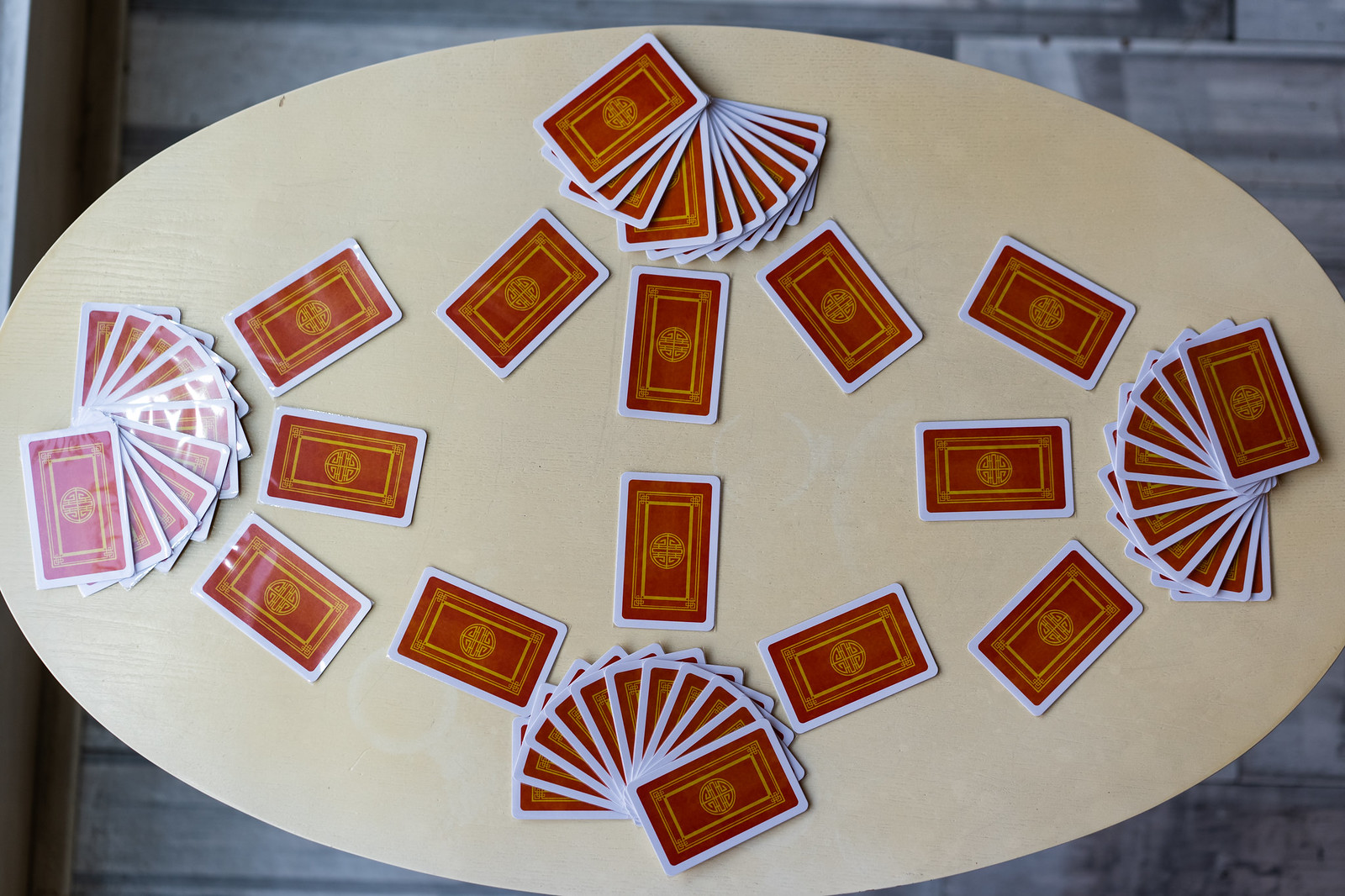The image depicts an oval-shaped table in a light wood finish, reminiscent of a whitish beige color. On the table are approximately 50 playing cards, arranged in a seemingly haphazard manner. Four hands of cards are distributed across the table, all face down, obscuring their identities. Interspersed among these are several more cards, almost evenly spread out in the center. The cards themselves feature white borders and a vivid mix of red and orange hues. The background reveals a gray wooden floor, adding contrast to the scene. Notably, the table is devoid of people, leaving the cards as the sole focus.